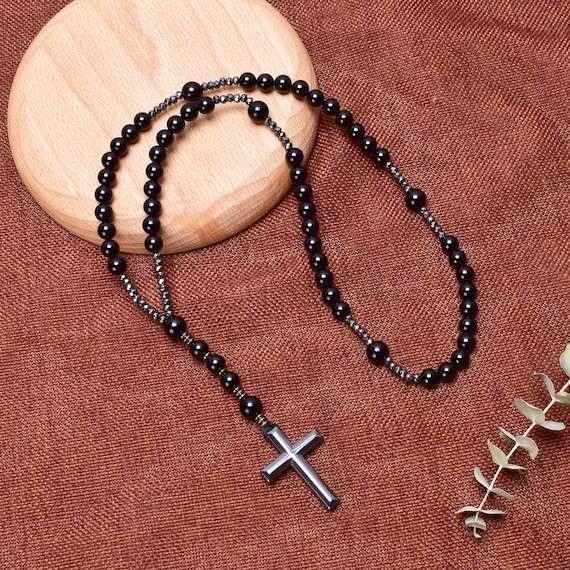This is a professional photograph showcasing a black beaded rosary necklace with a polished silver cross at the end, synonymous with Christianity. The necklace is artfully arranged on a gently sanded wooden disc, and the background features a brownish-red burlap cloth, providing a rustic but elegant contrast. The spherical beads of the necklace are glossy and smooth, with larger beads interspersed with smaller ones, looping in a traditional rosary design. To the bottom right of the image, a stem of dried plant with light green leaves subtly creeps into the frame, adding a natural touch. The composition suggests a carefully cropped photograph, potentially part of a larger image, aimed at highlighting and promoting the necklace.